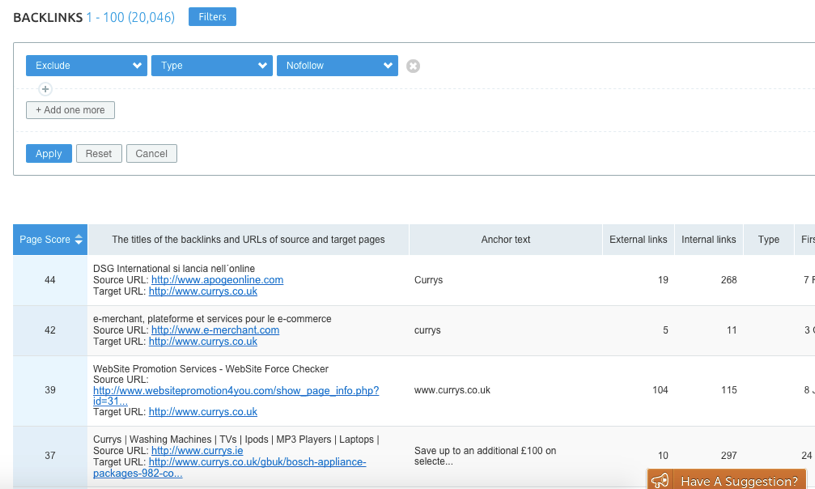This image depicts a web page designed for tracking backlinks, which are essentially links from other websites pointing to your own. 

At the top-left corner of the page, the headline boldly states "BACKLINKS" in black, capital letters. Adjacent to it, in blue font, is the text "1 to 100" followed by a dash and the number "20,046" in parentheses, indicating the total count. To the right, there's a blue rectangular button labeled "Filters."

Below the filters button, there are three filtering categories, each enclosed in a blue rectangle: "Exclude," "Type," and "No Follow." Beneath these categories is a gray box reading "Add one more," followed by blue text saying "Apply" and gray text saying "Reset" and "Cancel."

Further down, there is a listing of individual backlinks. The header for this list is gray and includes columns titled "Titles of the Backlinks," "URLs of Source and Target Pages," "Anchor Text," "External Links," "Internal Links," "Type," and a partially visible column on the far right with an unclear header that starts with "Fi."

The page displays four different listings of backlinks. The far-left corner of the image shows a sidebar with blue text listing numbers sequentially: 44, 42, 39, and 37.

Each section and filter is designed to help users easily navigate and manage their backlinks.